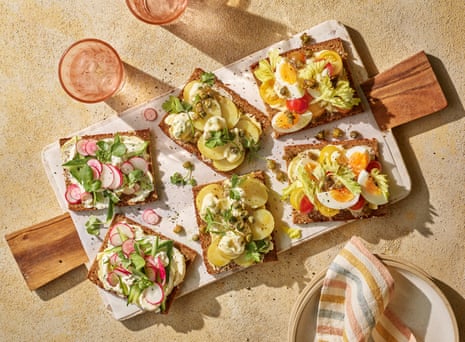This overhead photograph depicts a serene, summery picnic setting with a meticulously arranged serving board placed on a light tan, bisque-finished surface. On the board, which has a white rectangular center framed by wooden sides, there are three open-faced sandwiches, each crafted on brown or multi-grain bread and split into six smaller pieces. The sandwich on the far left features a slice of brown bread topped with vibrant red radishes, fresh green garnishes, and a creamy spread. The middle sandwich showcases sliced yellow pears, walnuts, and chopped greens, accompanied by a white dressing. The sandwich on the right combines hard-boiled egg slices, red tomato slices, and leafy greens. Flanking the board are two pinkish-hued glasses filled with ice water, adding a refreshing touch to the scene. In the bottom right corner, a small stack of plates is adorned with a folded striped linen napkin, displaying terracotta red, gold, and medium blue stripes, suggesting a warm and inviting atmosphere perfect for a casual outdoor meal.